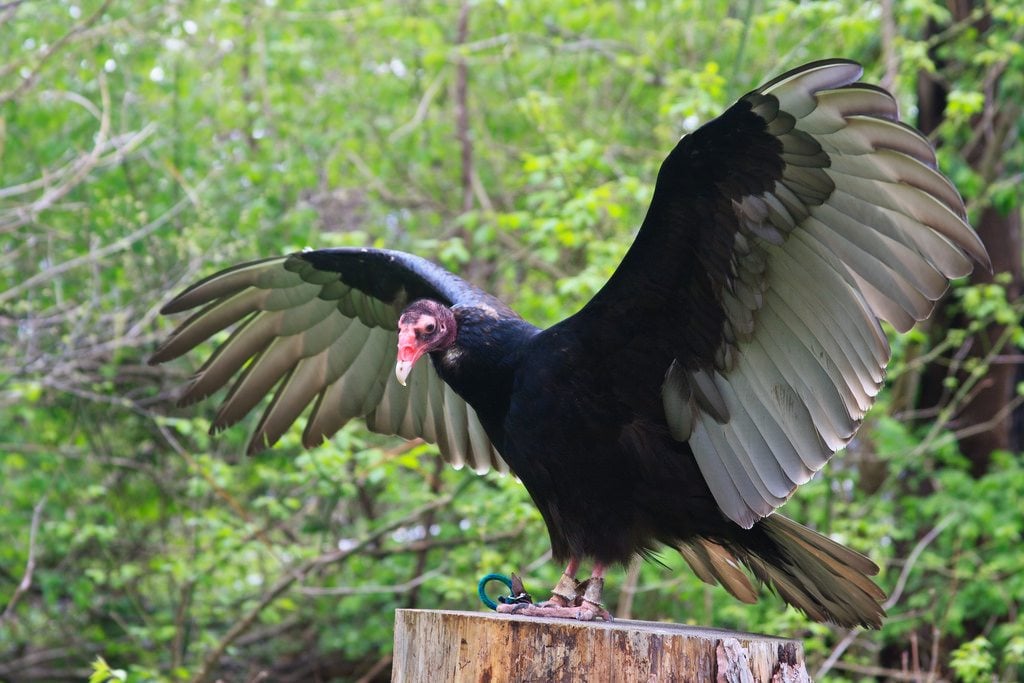The image features a striking turkey vulture standing on a tree stump with its wings majestically outstretched. The vulture's body is adorned with black feathers, while the undersides of its wings reveal a touch of white and gray near the base. Its tail feathers display a mix of black and cream. The bird's head is devoid of feathers, showcasing purple and pink skin, complimented by a large, hooked, white beak tinged with red. The vulture's feet are wrapped with leather bands, suggesting it might be in captivity, and are connected with a green string. Its legs have a slight reddish hue. The backdrop is a blur of trees, lending a natural yet indistinct background to the detailed portrait of this magnificent bird.